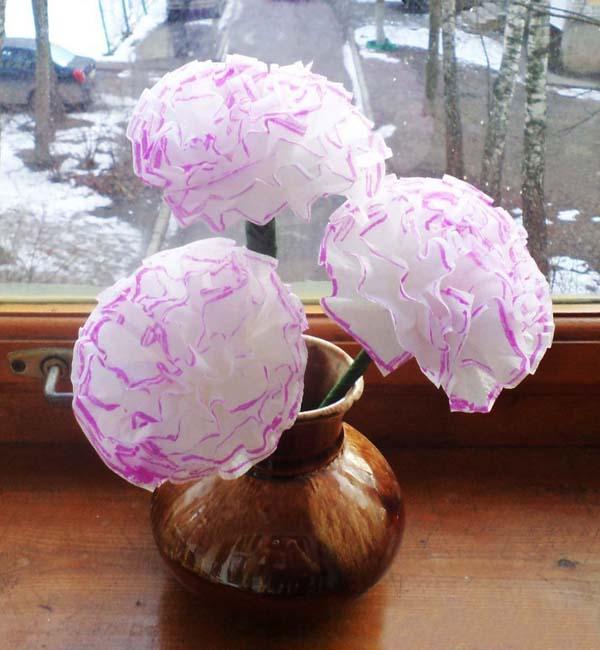This is a color photograph taken indoors, showcasing a handmade, brown ceramic vase placed on a wooden windowsill. The vase contains three large artificial flowers, which appear to be handmade from tissue paper or fabric. These flowers resemble carnations with mostly white petals that have purple edges and are supported by thick green stems. The center flower and the one on the right have visible stems, while the stem of the flower on the left is not as apparent. The wooden windowsill has a metal handle on the left side, and the bottom frame of the window is visible. Through the glass window, an outdoor winter scene can be observed, featuring a street with a parked car in the upper left-hand corner, a white building, visible stairs in the upper right-hand corner, some gray tree trunks, shrubbery, and patches of snow and ice covering parts of the ground.